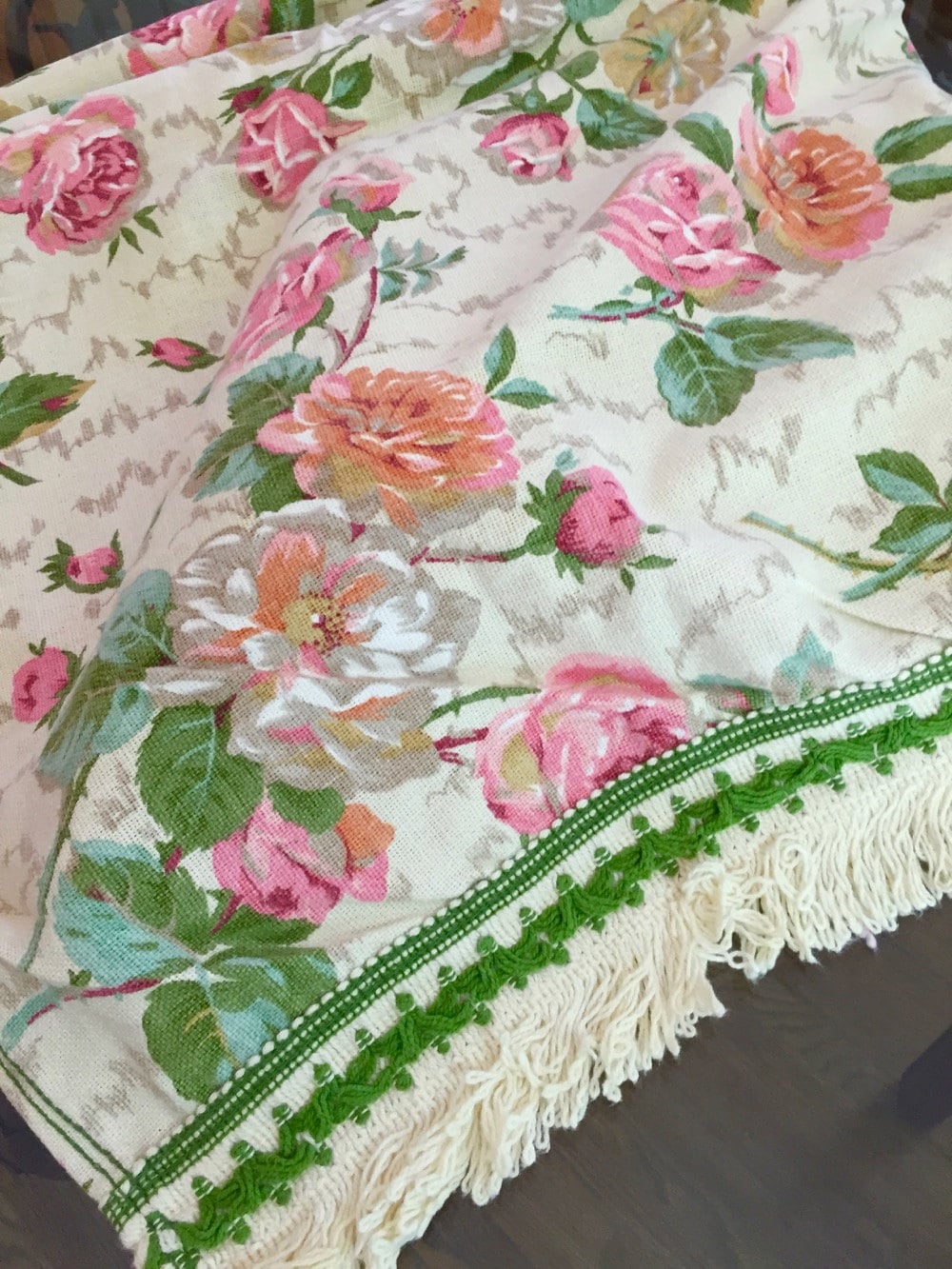The image features a beautifully detailed, hand-sewn quilt placed on a dark wooden surface, possibly a table or floor. This quilt showcases an elaborate design of clustered roses in shades of white, pink, and a hint of orange, each surrounded by lush green leaves and stems. The primary fabric of the quilt is cream-colored, with intricate grayish-brown squiggle patterns interwoven throughout. A striking green border with matching embroidery frames the quilt, complemented by a subtle cream fringe at the bottom. The quilt's material appears to be heavy and canvas-like, indicating a wide open weave. The richly ornate floral patterns on the quilt depict roses at various stages of bloom, adding to its textured elegance and handcrafted charm.